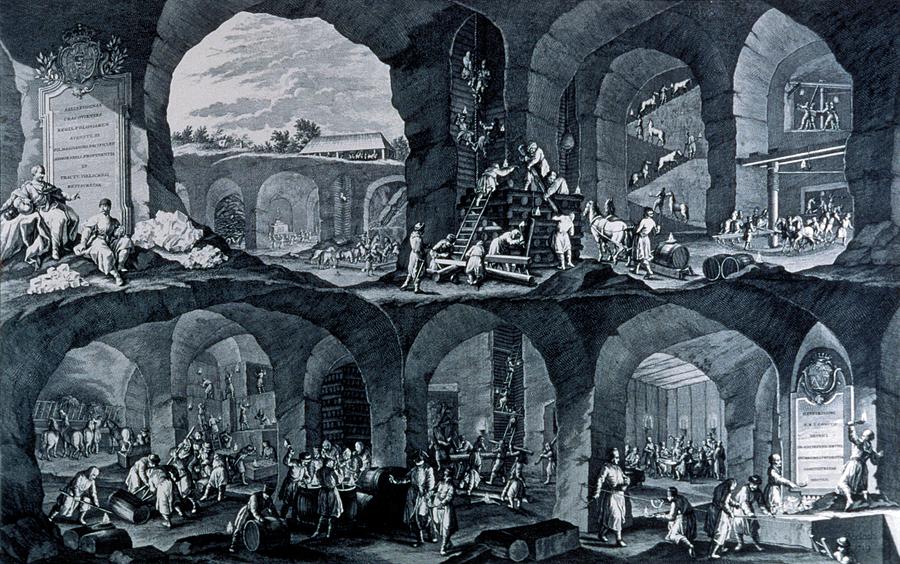The image is an intricate, black and white drawing that depicts a grand scene of industrious activity, potentially set in ancient Greece. The composition is divided into two distinct sections: an upper and a lower level. 

In the lower section, which seems to be underground, an elaborate network of archways dominates the scene. This area is bustling with dozens of people engaged in various forms of manual labor. Some individuals are seen pushing and pulling barrels, while others are mounted on horses or overseeing the work. Scaffolds and ladders facilitate the workers' movements within this space. Ornate statues adorn the walls, and a white plaque with inscriptions is visible on the right side.

In the upper section, which extends above ground, the activity continues with more people. This area features additional archways and a large staircase that many are seen climbing or working around. A large placard is affixed to one stone wall, near which a group of people are casually seated. The scene expands into the background where one can glimpse a cloudy sky and the roof of a building nestled among trees. The entire setup suggests a massive, epic-scale project, possibly an excavation or a monumental construction endeavor.